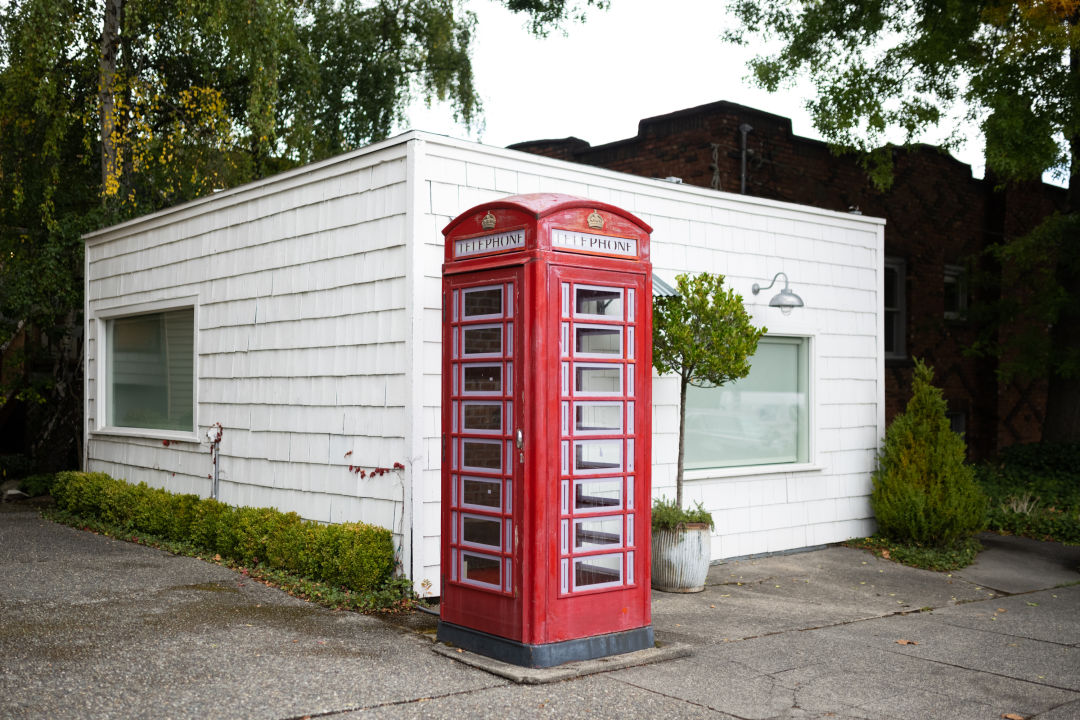A vintage red telephone booth stands prominently in front of a square white building, drawing immediate attention with its classic design. The booth features multiple glass panes with white frames along the sides, allowing glimpses through to the partially obscured doorway of the building behind it. Each side of the booth showcases a white signboard with the word "TELEPHONE" written in bold black text. 

The telephone booth itself is a rectangular red box set on a black base, which rests on a large stone platform surrounded by a stone ground. The booth's door has a small silver knob for access. 

The white building behind the booth has a flat roof and is constructed with rows of white wooden planks. Visible through the glass panes of the telephone booth, one side of the building features a window positioned on the left half, while the other side has a centrally located window with a lamp above it. Inside these windows, white curtains can be seen, adding to the building's simplistic, yet charming appearance.